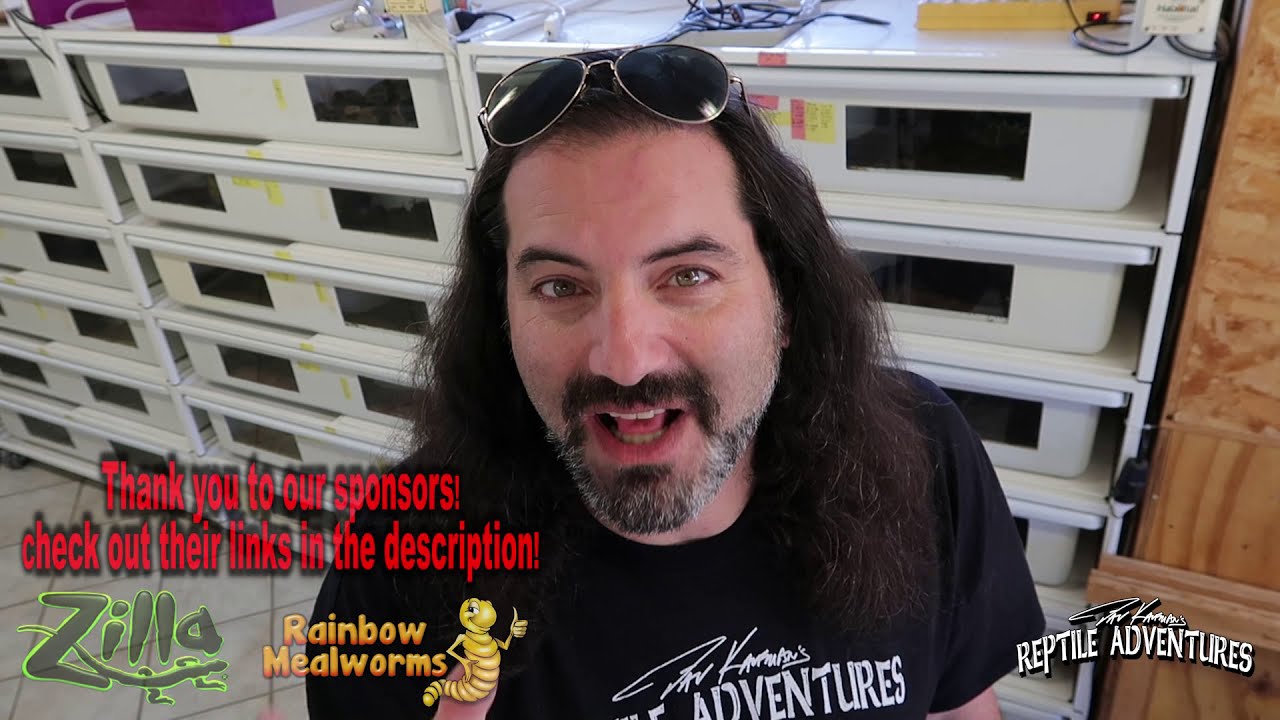The image depicts a man with a lighter skin complexion, long black hair flowing past his shoulders, and a short goatee beard. He is wearing a black t-shirt with the inscription "Reptile Adventures" and a signature above it. He also has sunglasses perched atop his head. The man is looking directly into the camera with his mouth open, seemingly in the middle of speaking, suggesting that the image is a screenshot from a video.

On the lower left corner of the image, the text "Thank you to our sponsors, check out their links in the description!" is displayed in red font. Beneath this, in black font with a green border, it reads "Zilla," accompanied by a design resembling a salamander. Next to it, to the right, is the phrase "Rainbow Mealworms" in yellow letters, alongside a cartoon image of a yellow mealworm with stripes and a thumb up. 

In the background, there are several white bins neatly organized within shelving units, and to the right, wooden cabinetry or drawers can be seen, adding to the structured setting.